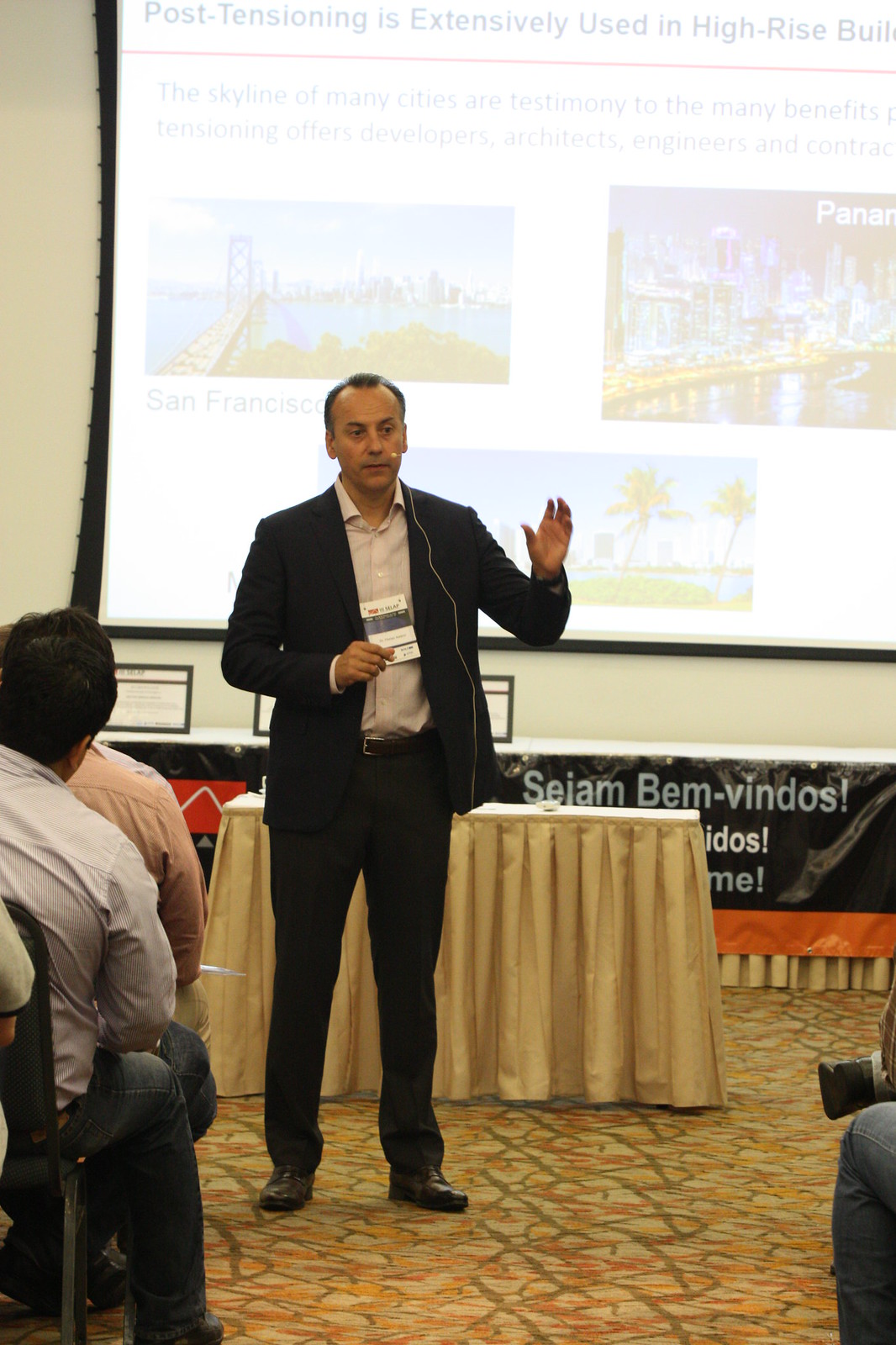In this detailed color photograph with a portrait orientation, a man stands at a conference, delivering a speech to an audience. He is dressed in a black suit with a white button-down shirt and is wearing an earpiece. His left arm is raised, emphasizing a point, while he holds a brochure in his right hand, positioned in front of his chest. His short black hair shows a receding hairline. The audience, partially visible, consists of at least four seated individuals, with only their backs and legs in view. Behind the man, a small table adorned with a gold tablecloth stands near a large projection screen. The slide on the screen reads, "Post-tensioning is extensively used in high-rise buildings," though "buildings" is partially cut off. Accompanying the text are three images: a bridge with a city in the distance, a cityscape at night, and a picturesque scene with palm trees, green grass, a lake, and a city in the background. The floor beneath him is a mix of yellowish-orange and brown hues, while the background wall is white, contributing to a clean and professional setting.